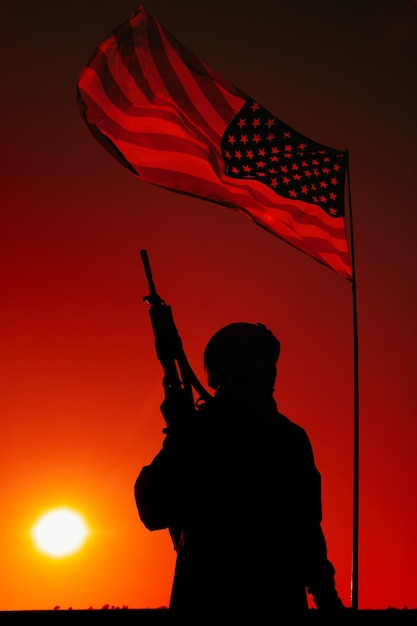A powerfully evocative image featuring a silhouetted soldier holding a rifle aloft, standing beneath a waving American flag. The silhouette, with distinct outlines of traditional battle dress and helmet, stirs patriotic undertones. Dominating the background is a dramatic sky infused with rich hues, transitioning from the fiery yellow and orange tones of a sun that appears to be either setting or rising, gradually deepening to a darker, brick red and almost black towards the top of the image. The American flag, rippling majestically in the wind, is notably tinted red by the intense coloration of the sky, lending a darkened appearance to the blue starfield while the stars and stripes remain distinguishable. The combination of these elements creates a striking contrast, highlighting the silhouette and the flag against the backdrop of a vivid, gradient sky, encapsulating themes of heroism, sacrifice, and national pride.